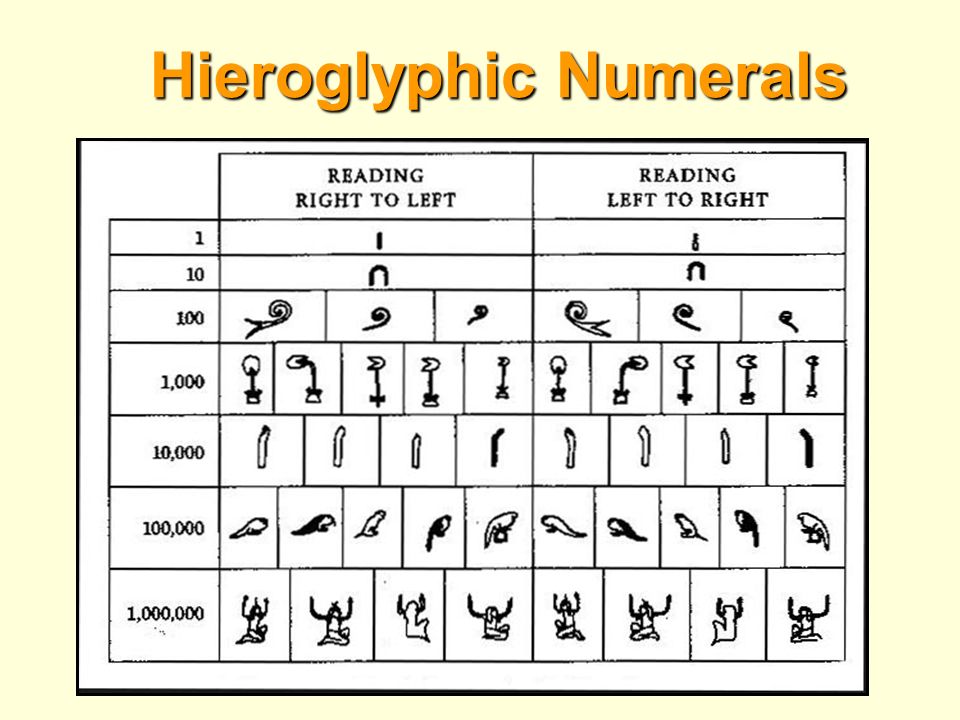The image displays a detailed chart of hieroglyphic numerals with a background in light yellow. At the top of the chart, an orange header with black outlines reads "Hieroglyphic Numerals." The chart itself is presented within a large white rectangle outlined in black. On the left side of the chart, a column lists the numerical values in ascending order: 1, 10, 100, 1,000, 10,000, 100,000, and 1,000,000, all written in black ink. The top row categories differentiate between "Reading Right to Left" and "Reading Left to Right."

The hieroglyphic symbols corresponding to each numerical value are displayed in two columns. The column under "Reading Right to Left" shows the hieroglyphic symbols oriented accordingly, while the column under "Reading Left to Right" shows the same symbols but mirrored. 

Specific examples of these hieroglyphic numerals include:
- 1: a single vertical line,
- 10: a horseshoe-shaped symbol,
- 100: a coil resembling a snail shell, sometimes depicted with or without protuberances,
- 1,000: a potted plant with a blooming flower, occasionally shown with the stem angling to the left,
- 10,000: a finger with a curvature at the top,
- 100,000: a man with both hands raised in the air,
- 1,000,000: an image resembling a god with outstretched arms.

This chart provides a comprehensive reference for understanding how ancient Egyptians represented different numerical values through hieroglyphics, highlighting the orientation differences when read in different directions.